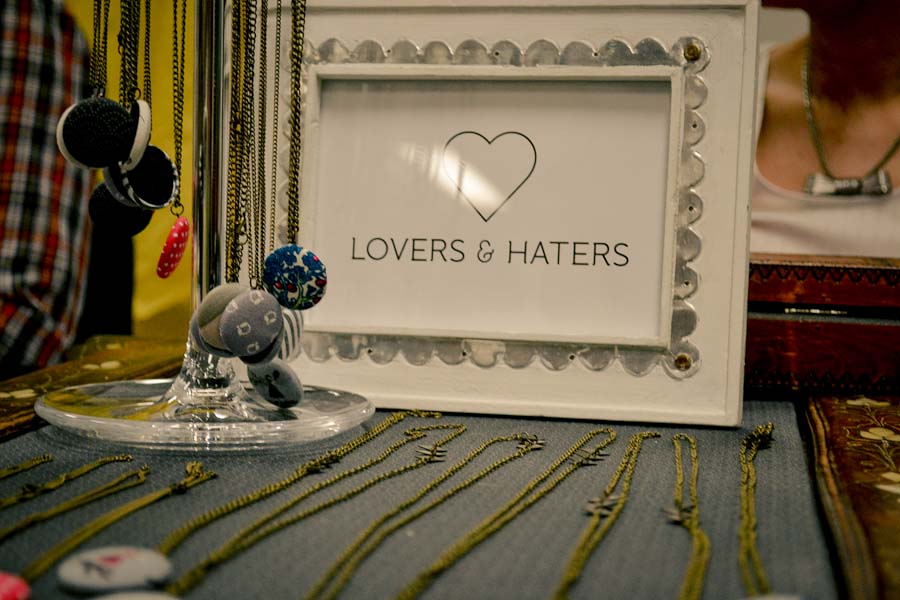The image is a detailed photograph of a jewelry display set against a backdrop of a white frame with silver beveling. Inside the frame, a simple black outline of a heart is depicted with the words "LOVERS AND HATERS" written in bold, all-capital letters. Centered in front of the frame is a clear plastic necklace holder showcasing various necklaces. These necklaces have distinctive buttons serving as medallions. The display is arranged on a gray matte surface with several gold necklaces laid out in front, creating a striking visual contrast. To the left, a clear tall pole extends out of the frame, with additional necklaces dangling from it. On the far left corner, a mirror reflects a person wearing a red and blue checkered shirt, adding a subtle human element to the scene. The image effectively captures the intricate details and careful arrangement of the jewelry and display elements.